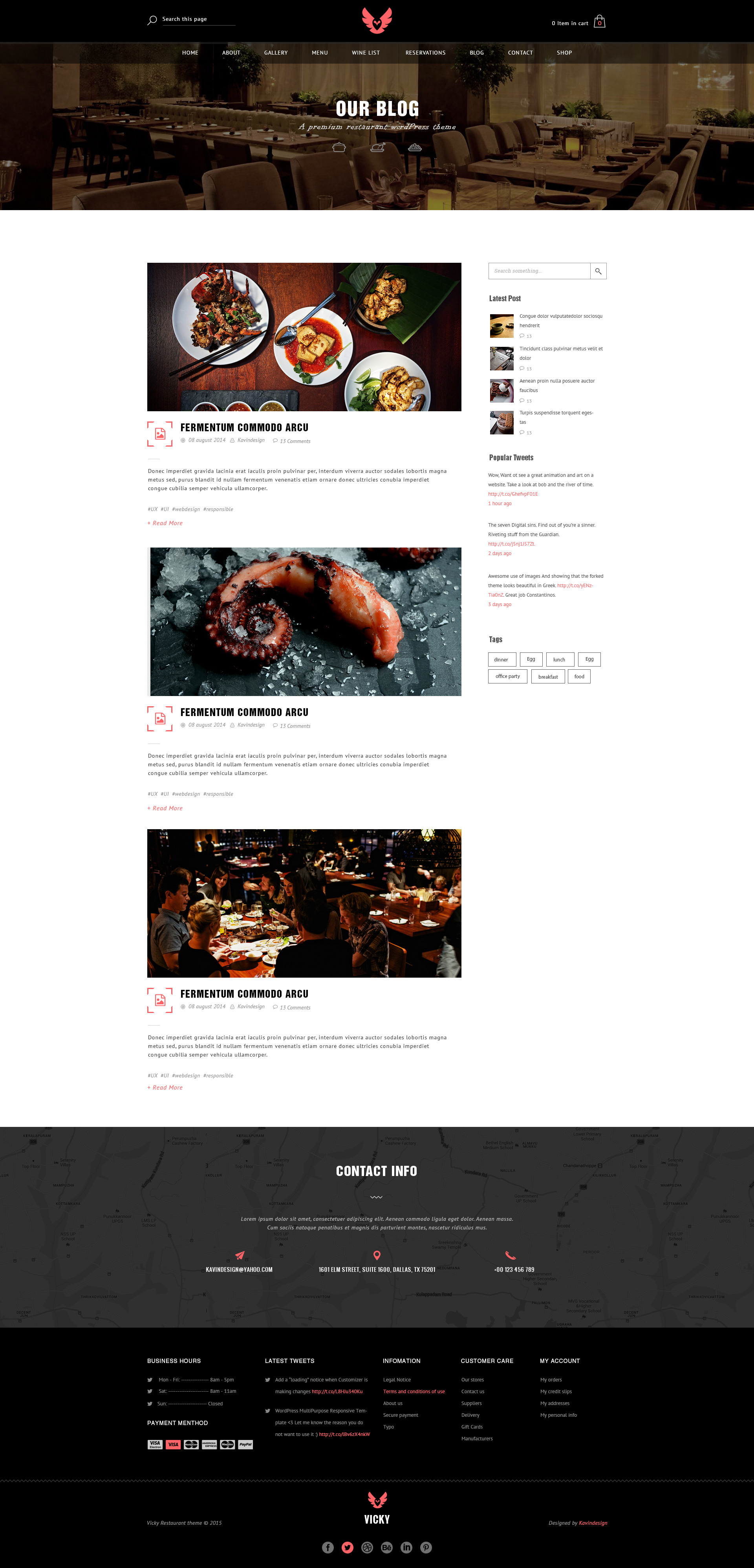The image depicts a webpage layout for a premium restaurant WordPress theme. At the top, the navigation bar includes links labeled "Home," "About," "Gallery," "Menu," "Wine List," "Reservations," "Blog," "Contact," and "Shop," with an empty shopping cart icon. The page prominently features a selection of food items, including an eye-catching display of octopus tentacles. Scrolling further down, the scene transitions to a bustling restaurant environment with patrons enjoying their meals. The footer of the page is marked by a black bar containing additional text and information.